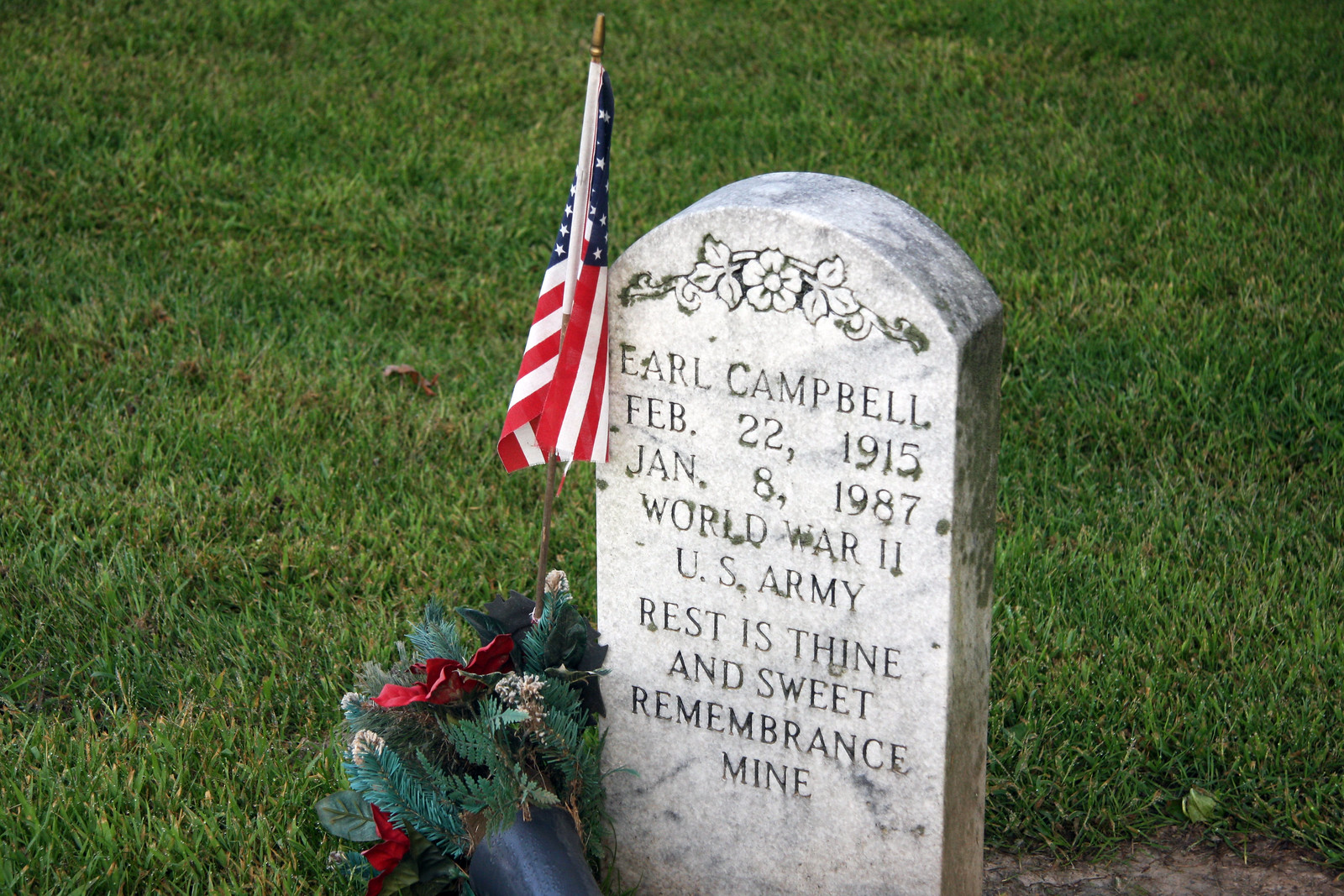Amid a tranquil cemetery setting, stands a weathered tombstone surrounded by lush green grass, subtly dotted with a few scattered leaves. The light gray marble or granite stone, aged with time and slight corrosion, prominently features a delicate flower design with trailing vines and leaves at the top. It marks the final resting place of Earl Campbell, inscribed with the poignant epitaph, "Rest in thine and sweet remembrance mine," detailing his life from February 22, 1915, to January 8, 1987, and honoring his service in World War II as part of the U.S. Army. To the left of this solemn monument, an American flag on a wooden stick leans respectfully, accompanied by an arrangement of artificial flowers at the base, and a small black pot that has tipped over. The daylight softly illuminates the scene, casting a gentle glow over this serene tribute.